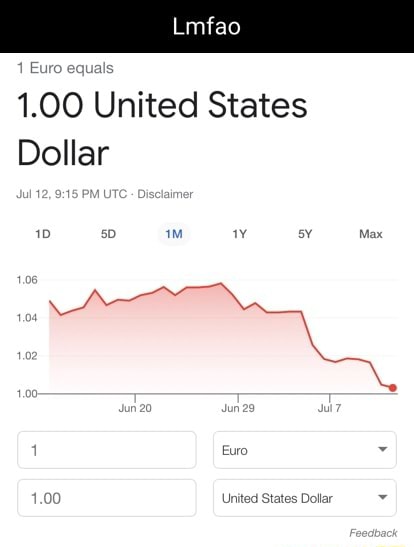The image features a black header strip with the text "LMFAO" displayed prominently. Below this, it states "One Euro equals 1.00 United States dollars - July 12, 9:15 p.m. UTC" followed by a disclaimer.

The main content of the image is a financial chart. Along the left side of this chart, there is a vertical scale starting at the bottom with values 1.102, 1.104, and 1.106. At the top, there are options for different time intervals labeled as 1D, 5D, 1M, 1Y, 5Y, and Max, with the "1M" option highlighted in blue.

The horizontal axis at the bottom of the chart is marked with dates: June 20, June 29, and July 7. The line plotted on the chart is red and fluctuates as it tracks the exchange rate over time. Initially, on June 20, the rate is around 1.05. It rises after about five days, then declines slightly, rises again briefly, and follows an upward trend before descending near the end of July. The highest point on the chart, approximately 1.06, occurs around June 27.

To the right side of the chart, there is a note stating "Feedback." The chart concludes with a value that shows the exchange rate has declined significantly by the end of the observed period, which spans more than a month.